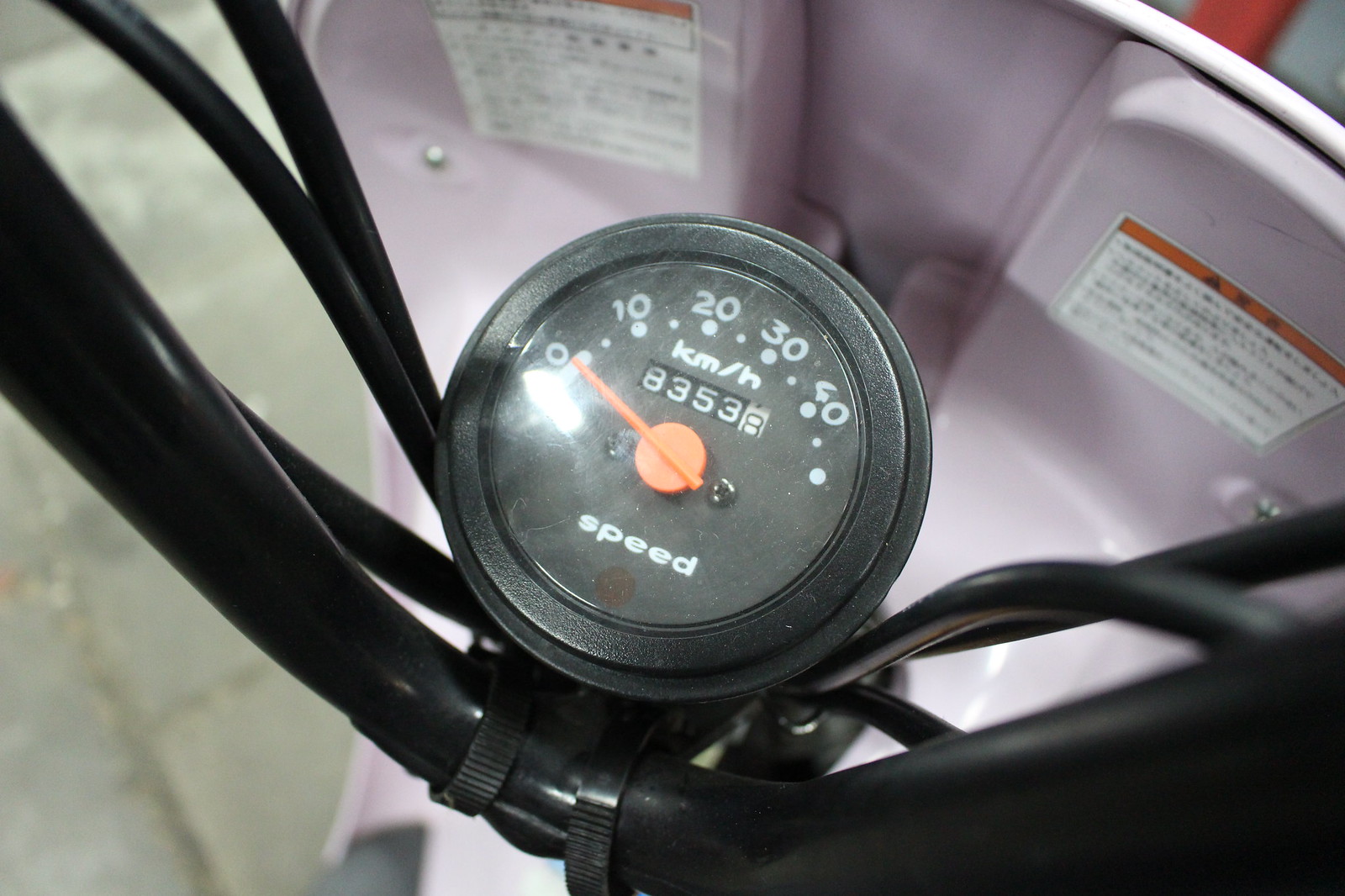A detailed caption for the image would be:

"A close-up view of an odometer with readings between 0 to 40 km/h and a total distance logged of 8,353,883,538 kilometers. The odometer is situated in an outdoor setting atop a surface made of concrete blocks or a concrete pad. Handlebars with brake wires extend from either side of the odometer, raising the question of why there would be brake wires on what appears to be a stationary object. In front of the odometer, there is a pink divider with writing and two warning labels on either side, enclosed in white squares with large tags written in an indecipherable language. The orange pointer on the odometer indicates a speed of 0 km/h."